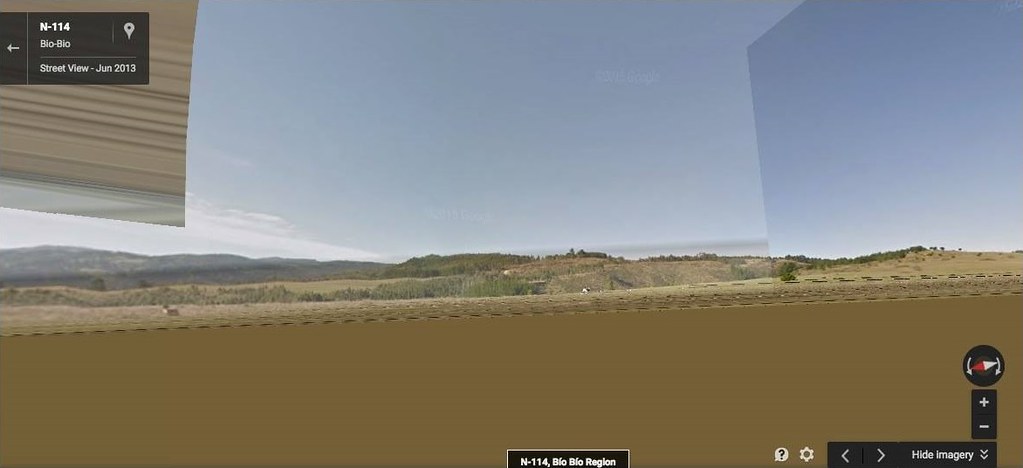The image appears to be a computer-generated representation, possibly from Google Maps or a video game, depicting a barren, desert-like landscape under a blue sky. The scene includes sparse vegetation and low, desert mountains that resemble dirt hills. In the upper left corner, text reads "N-114" with an unclear word below it, followed by "Street View, January 2018 or 2019" in small print. Another line says "BIOBIO," and below that "BIOBIO region." The bottom of the image features an interface with a tan bar, options for hiding imagery, a compass, and zoom controls (plus and minus signs) at the bottom right. There are also icons for a question mark, a gear, and arrows for navigation. A left arrow and map pin icon are present at the top left. The overall scene resembles a panoramic map view, blending elements of both real and simulated environments.